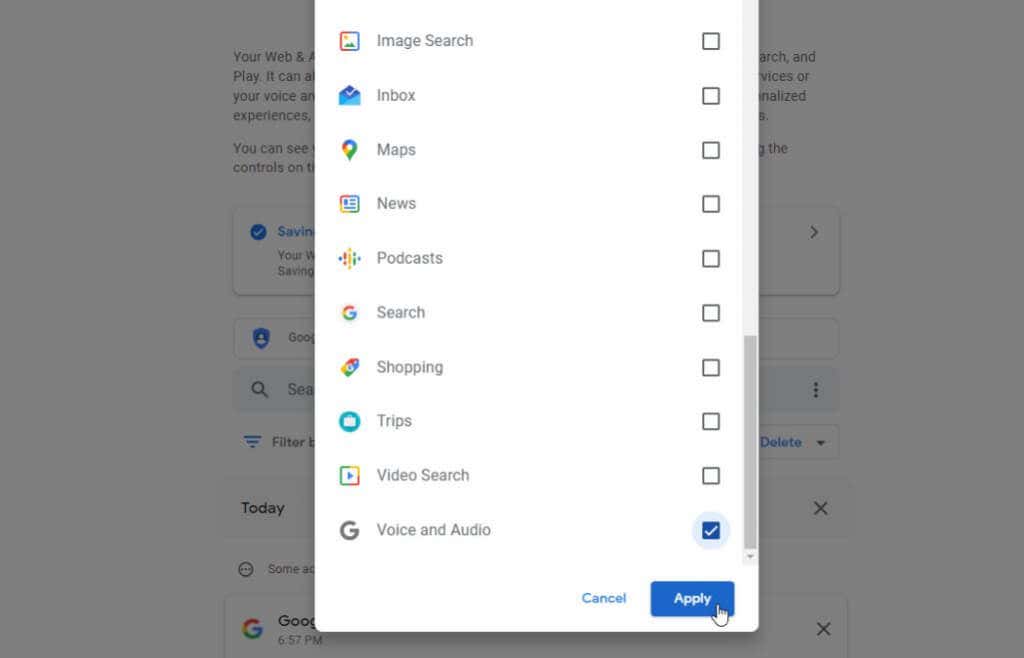The image depicts a smartphone screen displaying a gray background that is partially obscured by a pop-up window. The pop-up window is a white rectangle titled "Image Search," featuring a square icon on the left and a blank text box on the right. Below the title are several options, each accompanied by icons and checkboxes:

1. **Inbox**: Represented by a blue envelope icon with a checkmark box on the right.
2. **Maps**: Indicated by a dropped pin icon, with a blank checkbox on the right.
3. **News**: Shown with a square filled with lines, accompanied by a checked box on the right.
4. **Podcasts**: Depicted by colored lines next to a checkbox that is currently checked.
5. **Search**: Marked by a Google 'G' logo with a checkmark box to the right.
6. **Shopping**: Represented by a rainbow-colored price tag icon with an empty checkbox next to it.
7. **Trips**: Indicated by a circle with a white suitcase, and a blank checkbox on the right.
8. **Video Search**: Shown with a play button enveloped in a rainbow box, next to a blank checkbox.
9. **Voice and Audio**: Represented by a gray 'G' icon with a checkbox that is checked.

At the bottom of the pop-up, there are two buttons: "Cancel" and "Apply." The "Apply" button is blue and has a cursor hovering over it, indicating readiness for selection.